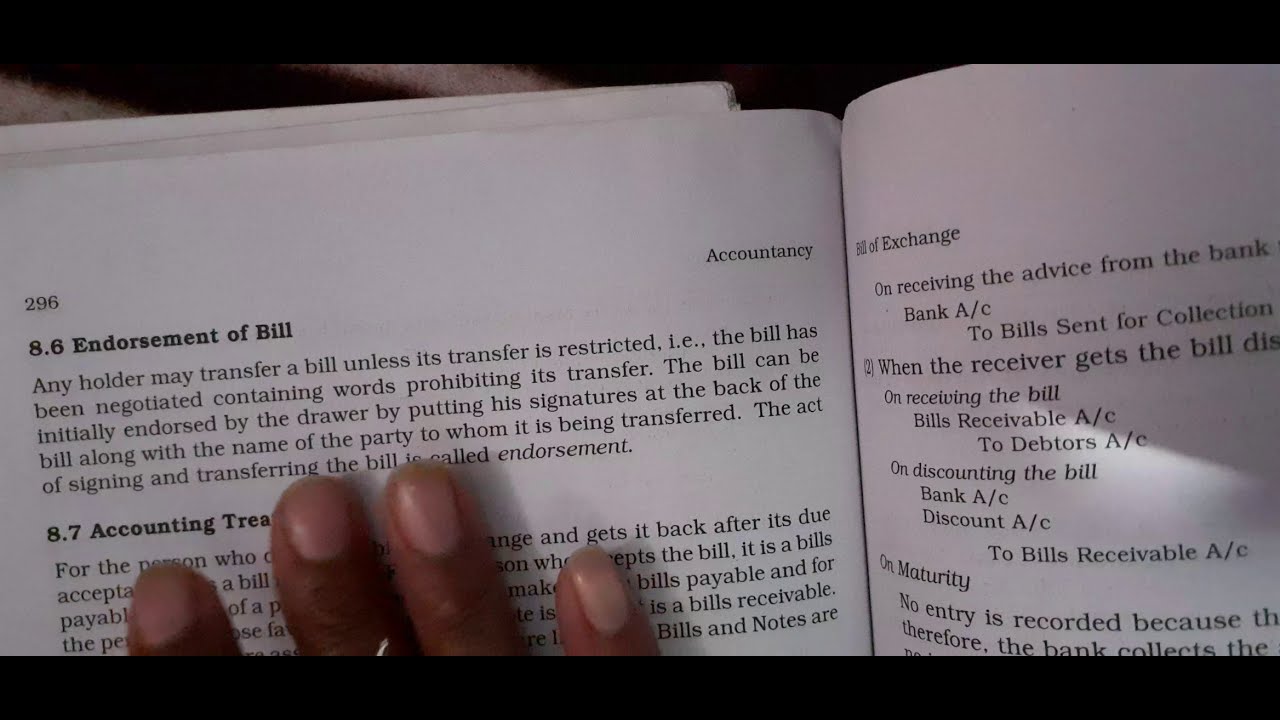The image is a wide, rectangular photograph showing the top portion of an open book. The photograph is cropped with black strips at the top and bottom. The book prominently displays the left page, numbered 296 in the top left corner, while the top right corner features the heading "Accountancy." Below the page number, the section titled "8.6, Endorsement of Bill" is visible. The initial text reads: "Any holder may transfer a bill unless its transfer is restricted, i.e., the bill has been negotiated, containing words prohibiting its transfer." The passage continues, introducing section "8.7" towards the bottom of the page. Four dark-skinned fingers, likely a woman's, cover part of the text on the left side, holding the page in place. The right page, though less visible, mentions topics such as "bill of exchange" and contains sections on "banking," "receiving a bill," and "discounting a bill," with a heading on "maturity" also present.